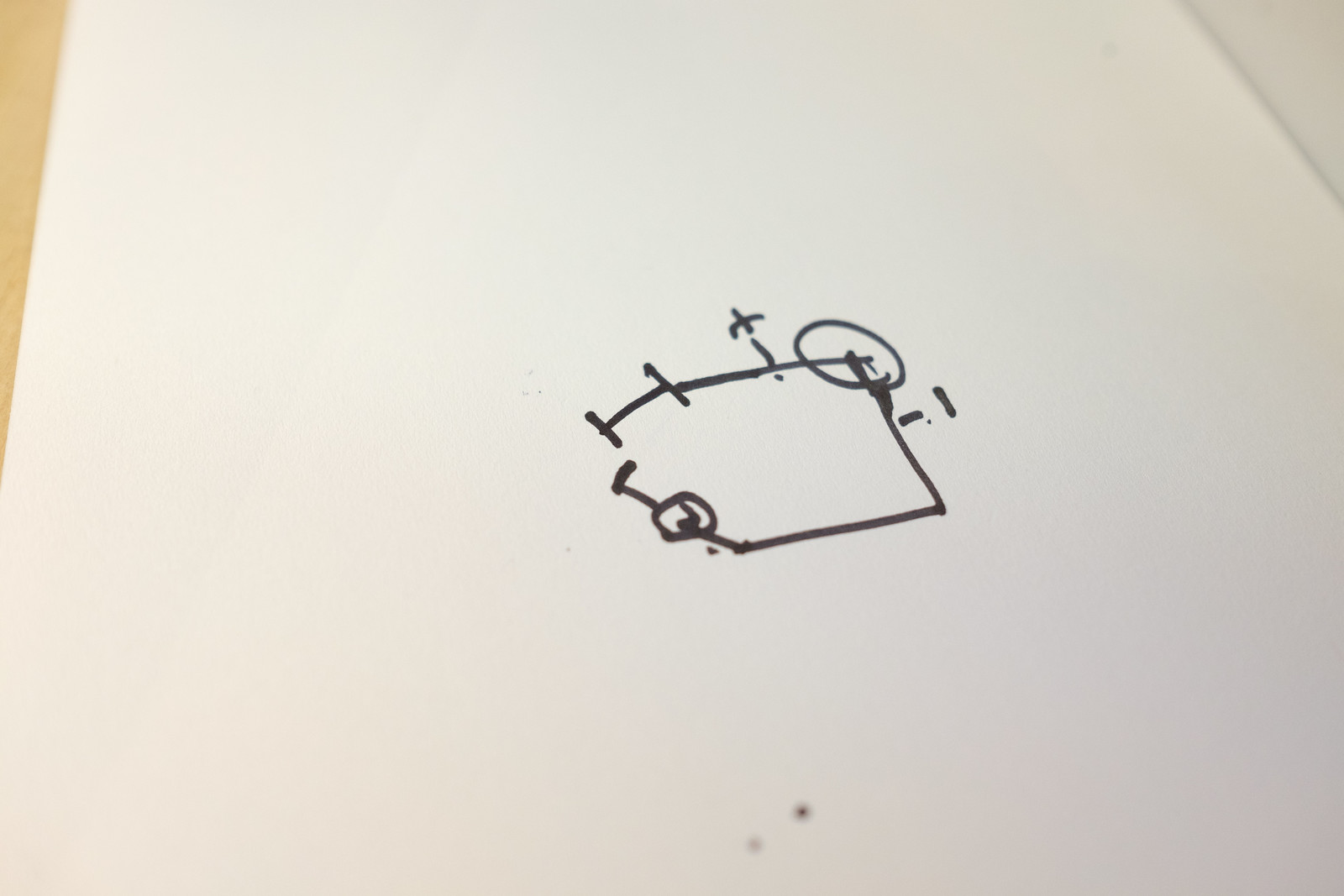In this image, a large piece of white paper features a small, intricate doodle created with a black marker, likely a Sharpie. The drawing includes a prominent circle situated on the right side of the paper. Emanating from the center of this circle are two lines. The upper line intersects with two additional lines, forming a T-shape near its origin. Additionally, there is another smaller circle, also with two lines extending from it, positioned nearby. Adjacent to these elements, a minus-one sign is visible, adding to the abstract complexity of the doodle. The overall shape of the doodle resembles a square with the left side missing, accentuating the incomplete, open-ended design. Below this primary sketch, two small black dots can be observed, contributing to the overall patterned appearance.